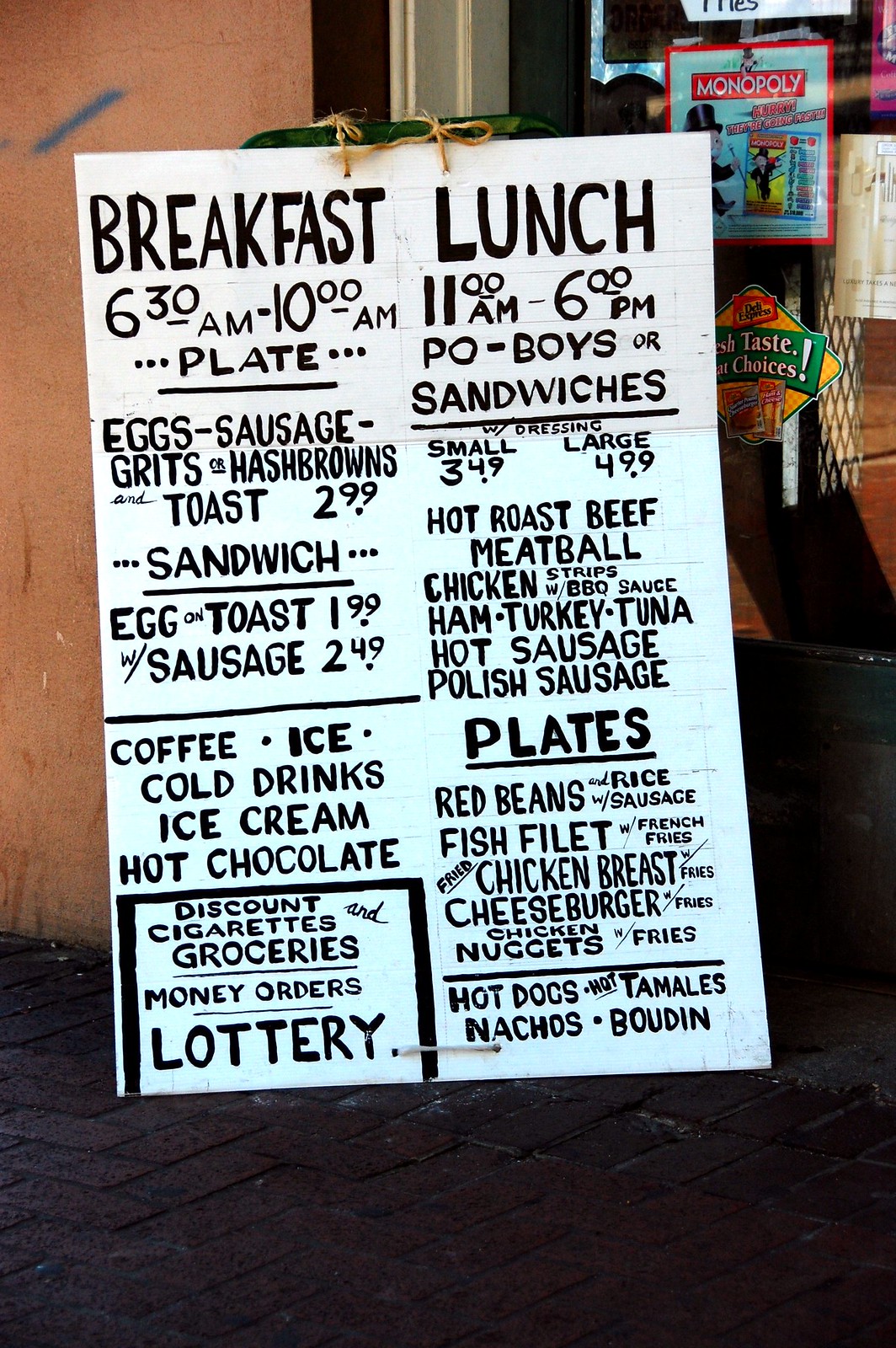In front of a bustling restaurant, a white poster board, meticulously handwritten in black text, details the breakfast and lunch offerings of the day. This sign is securely fastened with twine to a green, metal frame with elegantly curved edges at the top. The breakfast menu, served from 6:30 AM to 10:00 AM, features plates of eggs, sausage, grits or hash browns, and toast for $2.99. There's also a sandwich option: an egg on toast for $1.99, or with sausage for $2.49. Additionally, the sign advertises coffee, iced and cold drinks, ice cream, hot chocolate, discount cigarettes, groceries, money orders, and lottery tickets.

Adjacent to this, the lunch menu, available from 11:00 AM to 6:00 PM, lists an array of Po'Boys or sandwiches with dressing—small for $3.49 and large for $4.99—including options like hot roast beef, meatball, chicken strips with BBQ sauce, ham, turkey, tuna, hot sausage, and Polish sausage. They offer plates of red beans and rice with sausage, fish fillet with french fries, fried chicken breast with fries, cheeseburger with fries, chicken nuggets with fries, hot dogs, hot tamales, nachos, and the regional favorite, boudin.

Behind this informative board is a larger plywood panel positioned in the upper left corner, adorned with a spray-painted diagonal blue line. To the right, a window partially reveals a glimpse of the restaurant's interior, where brown wooden elements and possibly black metal or plastic features are visible. A prominent decoration on the window includes a Monopoly-themed sign, showcasing the iconic Monopoly man and a red rectangle with the Monopoly logo in white. Additionally, there's a smaller image of another Monopoly board featuring the Monopoly man. Below this, a diamond-shaped sticker with rounded edges is adhered to the window, displaying text that appears to read "Deli Express" at the top, in what might be black or blue text on a yellow shape within a red rectangle. The sticker continues with partially visible text that seems to say "Fresh Taste Great Choices!" on a green background.